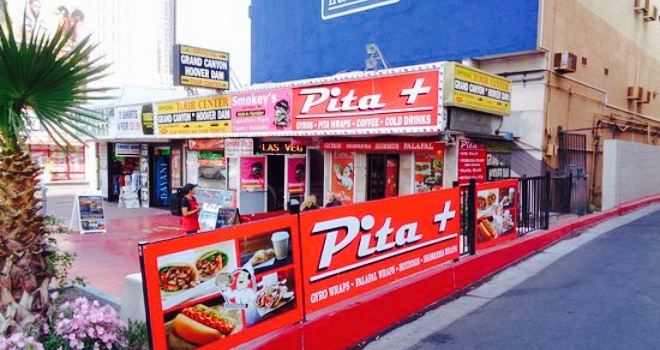The image depicts a vibrant city scene on a sunny day. Dominating the foreground is a small mom-and-pop shop named "PITA Plus," located off the side of a single-lane road marked with a white stripe. The shop is situated in front of a large tan building with a striking blue facade, which features pipes running down its right side. Between the building and the road stands a red fence adorned with an orange sign that reads "PITA Plus" in white text, along with pictures of various food items. Below the main text on the sign, blurred but partially legible, it lists offerings such as gyro wraps and falafel wraps. A smaller wall, approximately six feet tall, also extends in front of the building.

To the left, a palm tree with vibrant pink flowers at its base adds a touch of greenery to the setting. The courtyard area, featuring gray and red flooring, hosts a few individuals, including a person in a red shirt with a black baseball hat and knapsack. This individual appears to be observing the stores, enhancing the bustling yet cozy atmosphere.

Adjacent to the "PITA Plus" shop within the strip mall, there is a pink sign for "Smokie's" and another yellow sign with red print, decipherable only as "Tuer Center." Overhead, a sign promoting "Grand Canyon Hoover Dam" can be seen. The entire scene is framed by the diverse elements of urban life, with a compelling blend of colorful signage, greenery, and activity.